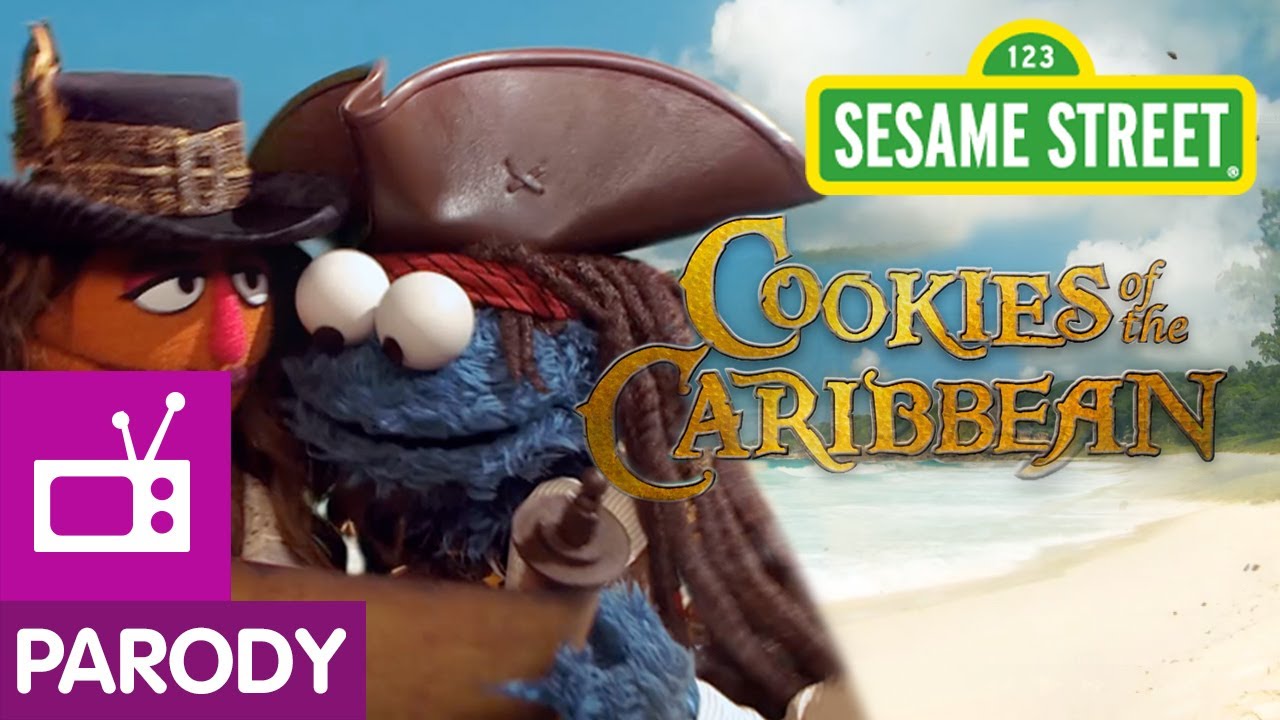The image is a parody-themed advertisement for "Sesame Street" with a whimsical twist inspired by "Pirates of the Caribbean." In the upper right-hand corner, the iconic Sesame Street logo is prominently displayed, featuring the familiar "123" in bold yellow, green, and white colors. Below this, in a font reminiscent of the "Pirates of the Caribbean" movie title, it reads "Cookies of the Caribbean," signaling the playful take on the popular franchise.

On the left side of the image, the Cookie Monster is humorously dressed as a pirate. He dons a brown leather pirate hat, complete with dreadlocks and a red bandana, and instead of wielding a sword, he holds a pastry roller. Alongside him is another recognizable Sesame Street character, an orange figure with a red nose, who wears a black pirate hat with a feather. The duo appears to be examining an unrolled treasure map, adding to the adventurous scene. 

In the background, a serene beach setting is depicted with a stretch of sand, a blue sky dotted with white clouds, and the ocean gently lapping at the shore. A small hill with green bushes adds to the picturesque landscape. Adding to the overall parody theme, a purple logo in the bottom left corner features a white outline of a TV next to the word "Parody" in white letters, ensuring viewers understand the light-hearted, comedic nature of the ad.